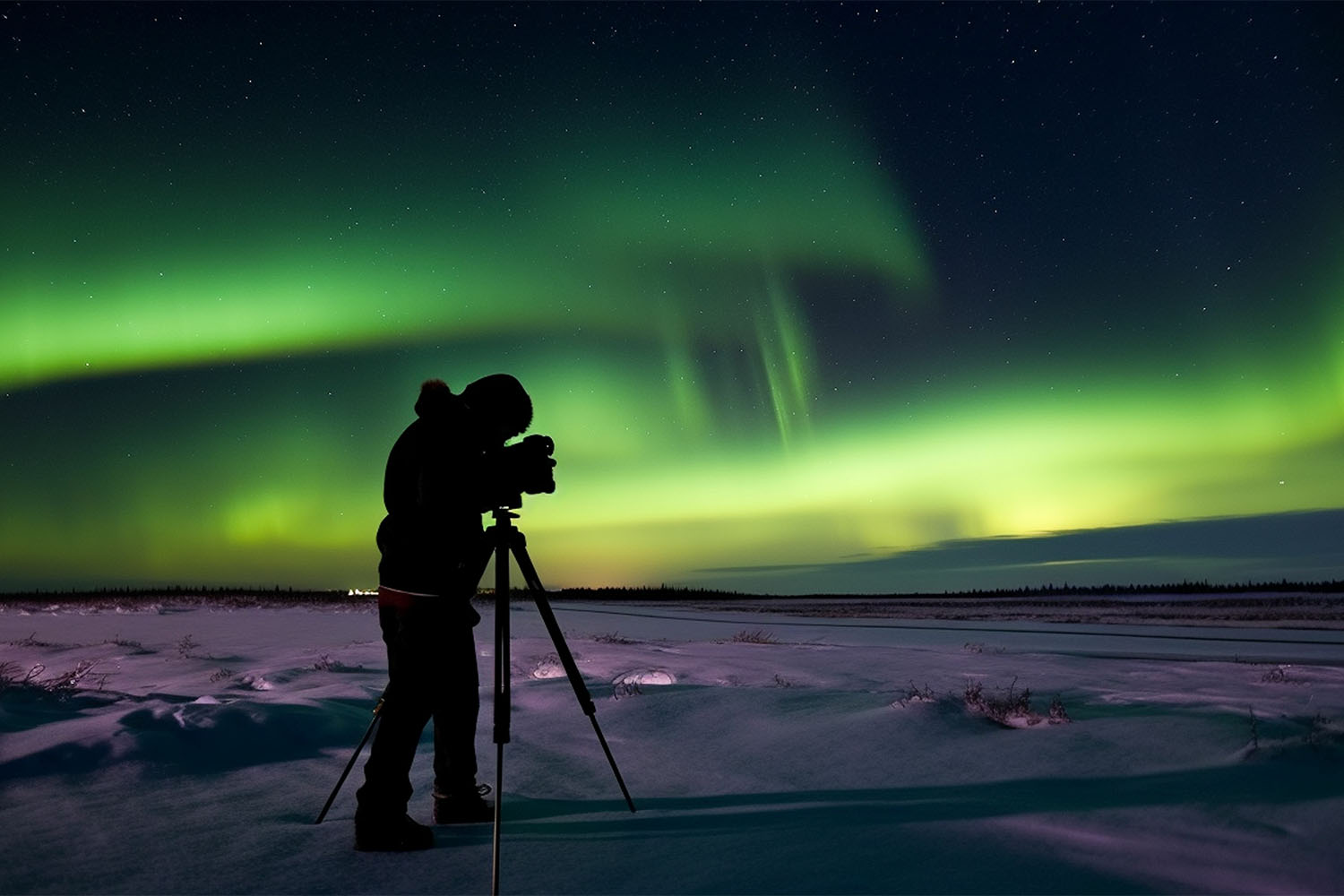This high-definition image captures a nighttime scene of a photographer silhouetted against a vibrant, snow-covered landscape. The man, dressed in pants and a jacket, is setting up his camera on a tripod, aiming to capture the stunning Aurora Borealis dancing across the sky. The aurora displays an array of vivid colors, predominantly green with hints of yellow and white, illuminating the star-filled sky. The snow on the ground, bathed in the aurora's light, takes on an almost otherworldly lavender or purple hue. In the distance, faint lights suggest a distant city or structure. Adding depth to the scene, the landscape features what appears to be a mountain range or elevated land on the horizon. The overall composition, with its rich contrasts and vibrant colors, might evoke the impression of being a computer-generated image, yet it captures the ethereal beauty of a cold, starry night under the aurora.